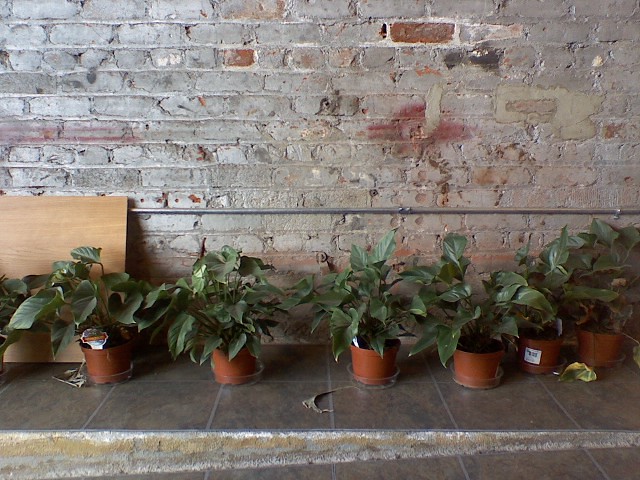In this detailed image, we're presented with an off-white brick wall featuring hints of grey, brown, and a touch of red brick seeping through, evoking a sense of aged charm. A grey metal pipe runs horizontally along the wall, positioned just above the height of the plants. On the far left, a light brown board leans against the wall, adding to the rustic atmosphere.

In the foreground, six terra cotta-colored pots, bearing a light reddish-brown hue, are arranged uniformly. Each pot is home to similar green leafy plants, all of which lack flowers and have large, teardrop-shaped leaves. The pots rest on a dark grey tiled surface, which appears slightly worn and discolored, suggesting it may have endured spills or rust. A lip of light brown and silver tile runs along the front edge of the floor, which seemingly transitions towards another similar dark grey tiled area, possibly indicating a slight ramp.

Overall, the scene captures a subtle blend of natural and industrial elements, underscored by the aged, yet vibrant, juxtaposition of bricks, metal, wood, and greenery.